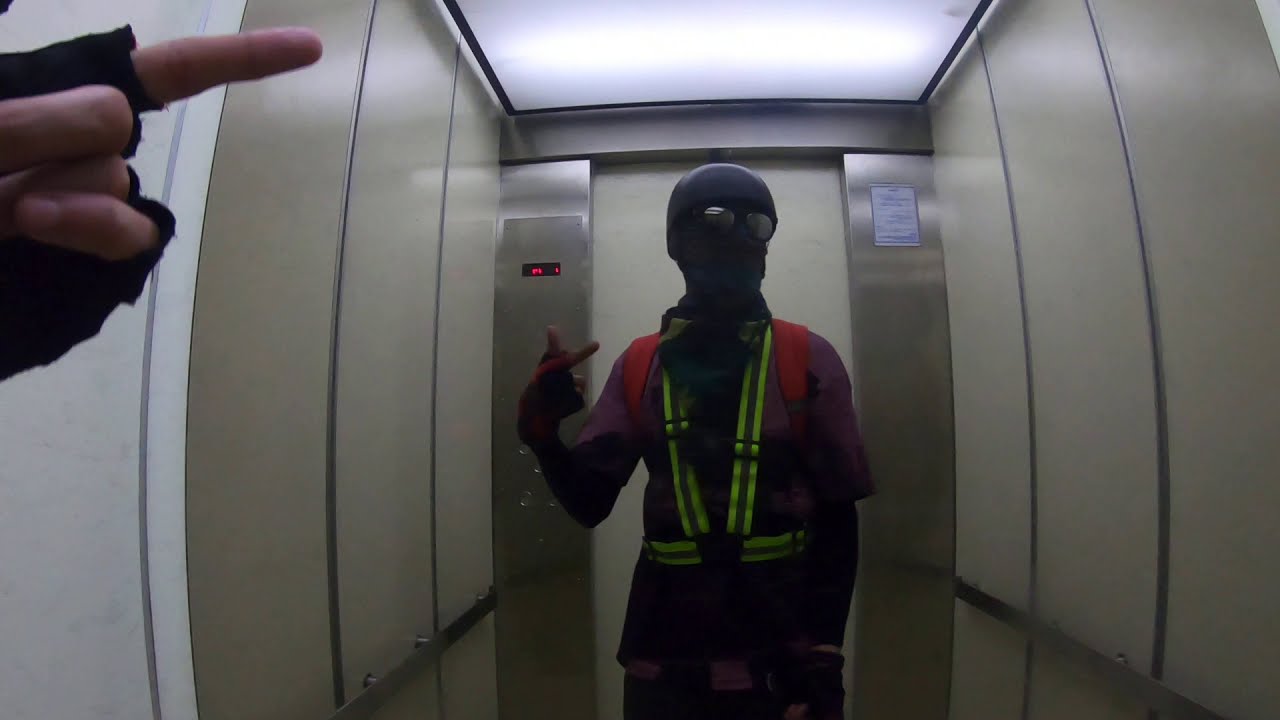The image portrays the interior of an elevator with beige walls and a fluorescent light at the top. At the center stands a man wearing a distinct outfit: a black helmet, black sunglasses, and a black mask, which partially obscures his face. His attire is a combination of red and purple, accented by a neon green belt around his chest and waist. Over his torso, he wears a reflective harness, and he has red backpack straps visible. His gloves are a mix of red and black, fingerless at the tips. He appears to be pointing to the left side of the elevator, although there is ambiguity in the gesture, as it could be misconstrued as giving the middle finger. In the top left of the image, a hand wearing a black glove with exposed fingers is pointing, adding to the illusion that this might be a mirrored photo, with the photographer's gloved hand visible both in reality and reflected.